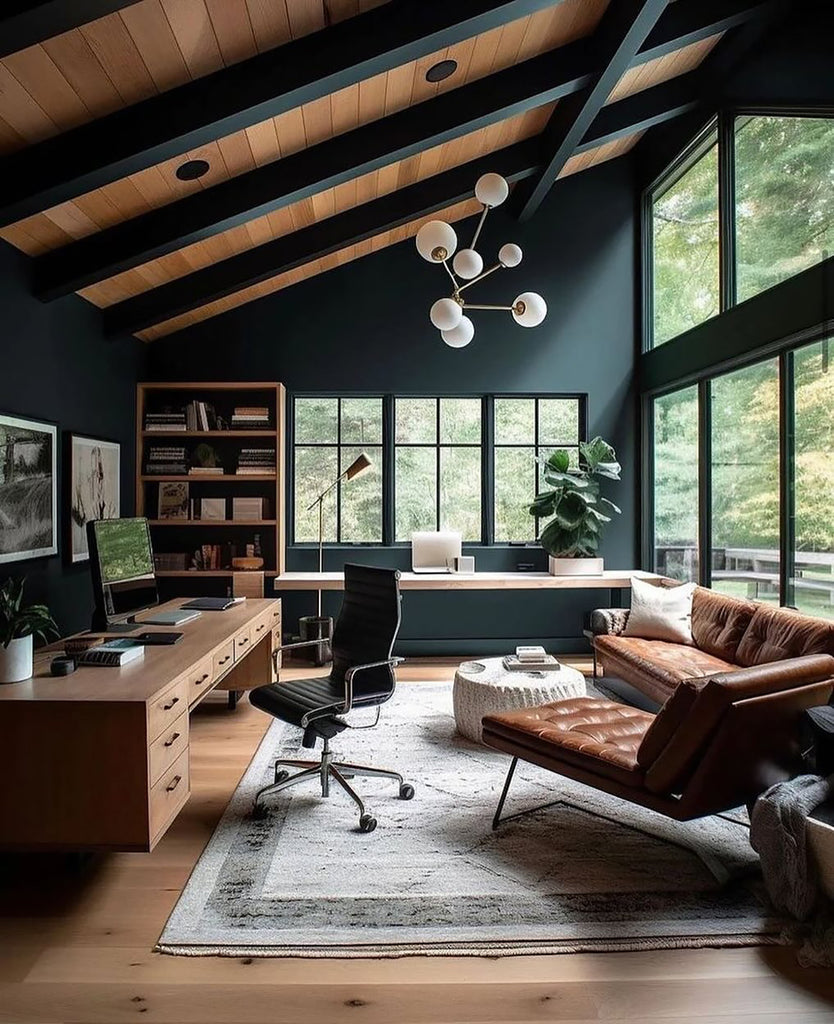This photograph depicts a sophisticated home office with a contemporary design and natural aesthetic. The room features a high-pitched cathedral ceiling lined with light brown wooden panels and accented by black beams. The floor appears to be light wood, possibly knotty pine or oak, and is partially covered by a large white area rug with a gray border. 

On the right side of the room, floor-to-ceiling glass windows, complemented by upper skylight windows, flood the space with natural light. Positioned against these windows is a brown leather sofa with a white throw pillow, accompanied by a matching chaise lounge angled towards the back wall. In front of the sofa sits a round white coffee table.

The dark slate gray back wall is adorned with three vertically aligned windows framed in black, and to the left stands a tall wooden bookcase. Against this wall, a long tan desk with multiple drawers and a light wood surface is neatly arranged with desk accessories, including a flat-screen computer monitor, a potted plant, and a desk lamp. Beside this desk, a high-backed black office chair with a silver metal frame and caster wheels offers a practical seating solution.

The overall color palette and arrangement of furniture—ranging from the brown leather seating to the sleek, functional workspace—create an inviting, yet professional atmosphere. The addition of framed paintings on the left wall and various office essentials underscores the multifunctional nature of the room, making it an ideal setting for both work and relaxation.